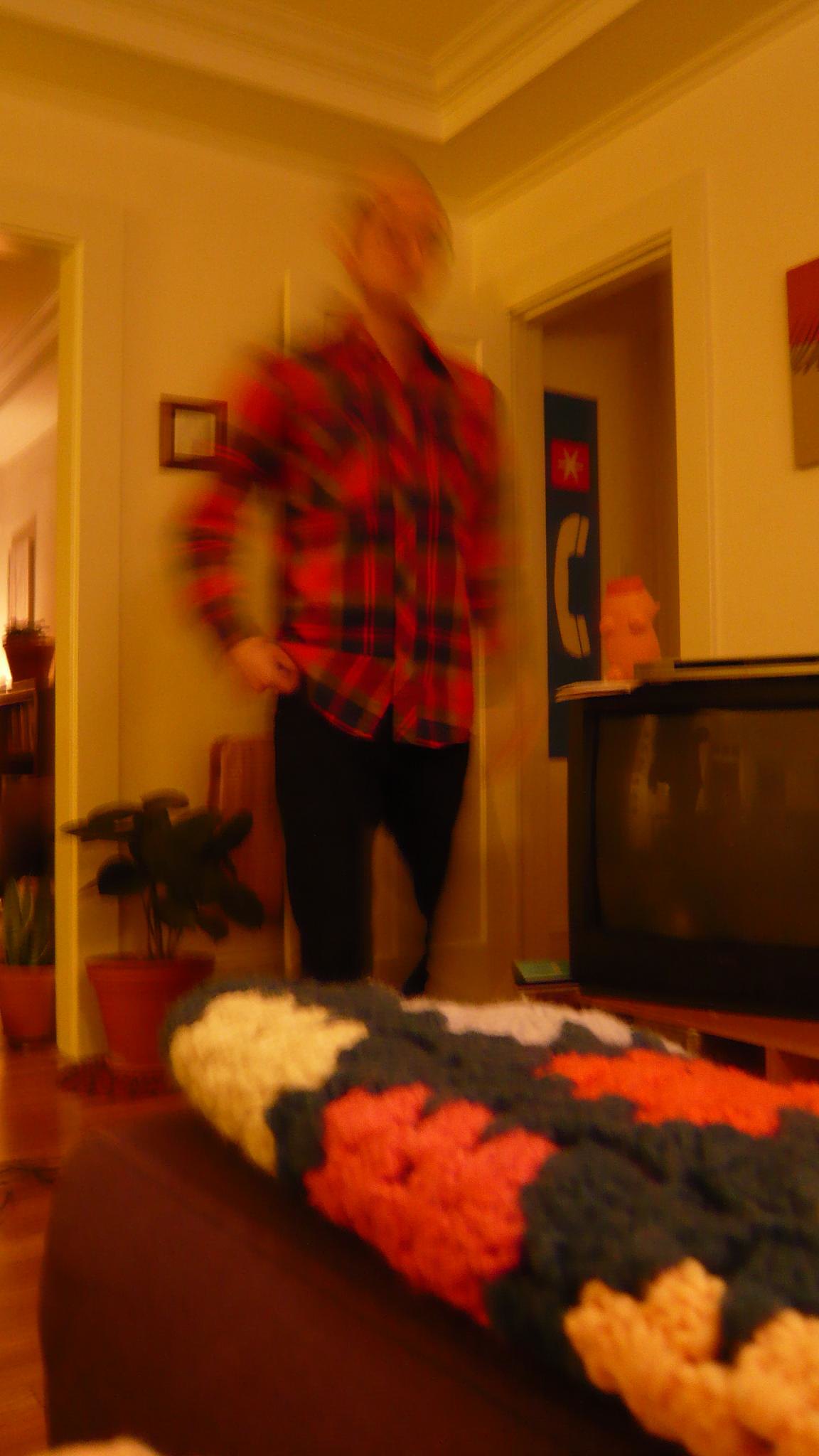A haunting photograph captures a living space, featuring a person standing slightly out of focus. The individual seems to exhibit a ghostly double exposure, with a blurred effect that makes parts of their body appear as though they are vanishing—reminiscent of the disappearing limb effect from "Back to the Future." Clad in a red and black flannel long-sleeve shirt paired with black pants, the figure stands against yellow walls. On the left and right, two doorways frame the scene, with the right door sporting a black sign emblazoned with a phone icon. In the background, a brown planter cradles a vibrant green plant, while an old black tube-style television sits to the right of the person. The foreground features a brown coffee table or ottoman, adorned with a woven quilted blanket in shades of black, yellow, green, and orange, adding texture and warmth to the mysterious setting.